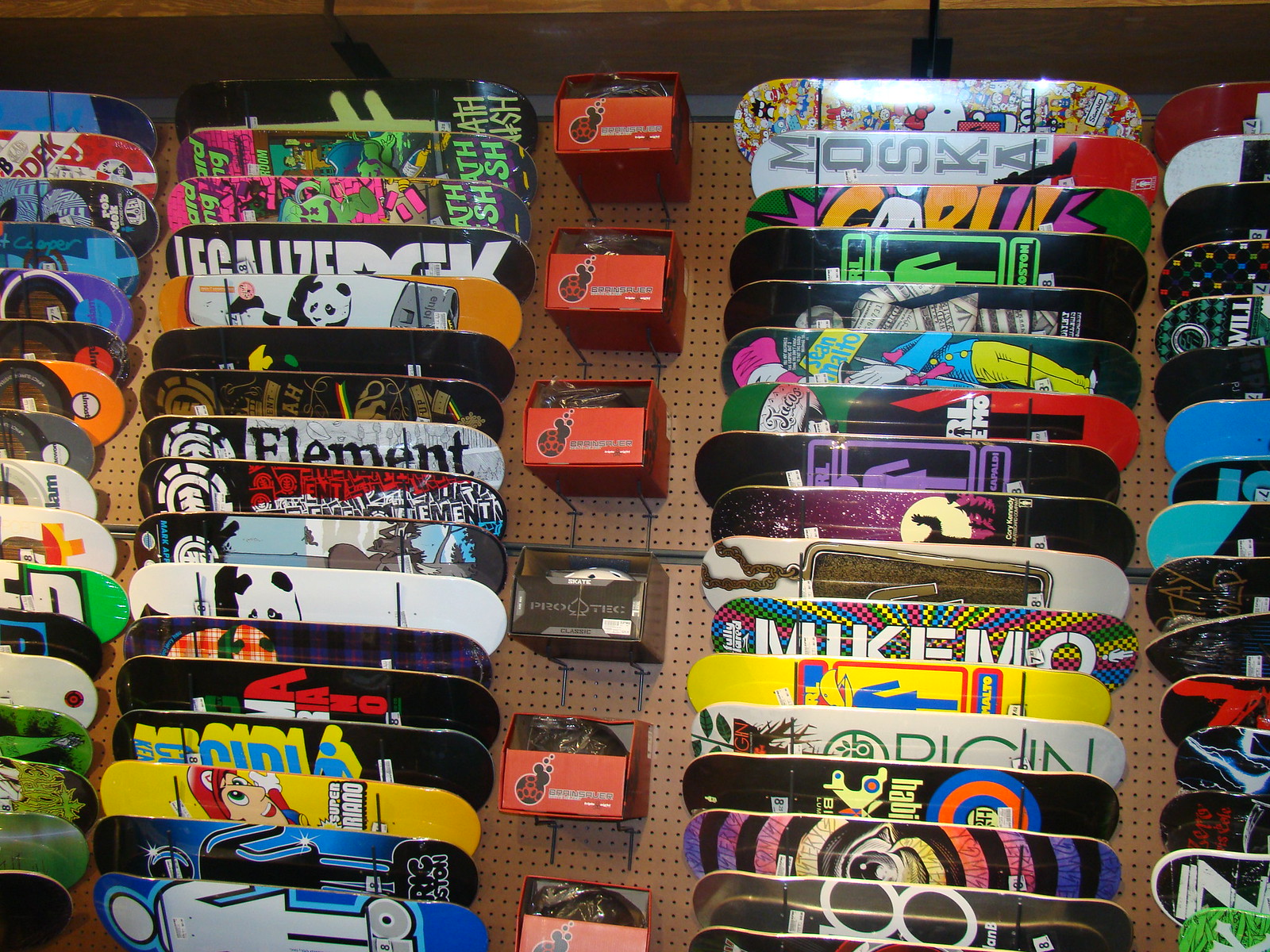This realistic photograph, horizontally oriented, captures the vibrant inside of a skateboard shop. The backdrop features a brown wooden pegboard wall with multiple holes designed for display cases and a matching overhang at the top. Dominating the center of the image are small red boxes interspersed with a single black box, presumably containing skateboard accessories such as wheels or helmets.

The main attraction on the left and right sides are the skateboard decks, arranged vertically in stacks. There are approximately four columns of decks, each holding 15 to 20 boards. Each deck showcases unique and colorful designs; some are adorned with graphic art, others with brand names. Notable designs include a white and black panda, the word "Element" in black text, and a variety of colors like red, yellow, black, and green. Other decks feature themes such as graffiti art, an eyeball with stripes, and even a Super Mario motif. This diverse array highlights the personalized nature of skateboard art, offering buyers a multitude of styles and brands to choose from.